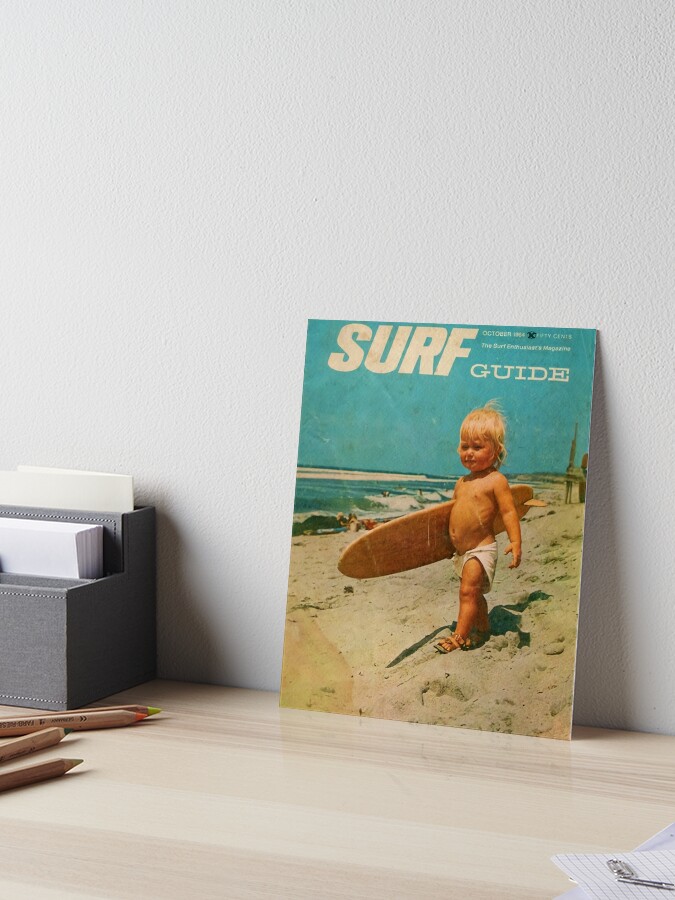This photograph captures a vintage edition of the "Surf Guide" magazine, which appears weathered with stains and signs of age. The cover features a white, androgynous toddler, perhaps around two years old, with very light blonde hair. The child is sans shirt, with either white shorts or a towel around their waist, and wearing sandals, holding a moderately large surfboard, relatively large compared to their small frame. The backdrop of the image on the cover illustrates a sandy beach with surfers and rough waves in the distance.

The "Surf Guide" magazine is propped casually on a light blonde wooden desk, leaning unstably against a neutral gray wall. The desk itself is cluttered with various stationery items: colored pencils, some loose papers, a small gray filer, and the corner of a notebook peeking into the frame. The overall ambiance suggests a casual yet nostalgic display, likely aimed at invoking a sense of laid-back, vintage surf culture.